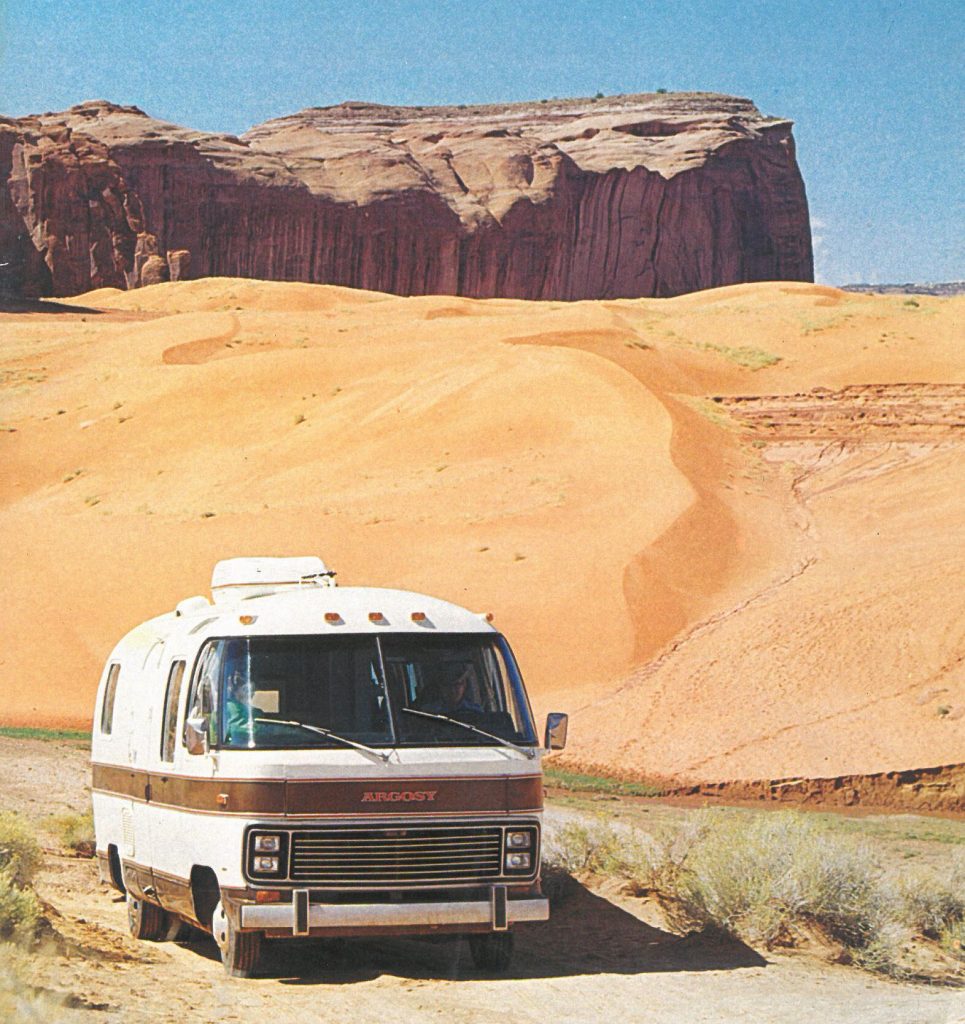The image depicts a desert scene with a vast expanse of sand under a clear, blue sky. In the foreground, a dirt road lined with sparse weeds and tumbleweeds cuts through the sandy landscape. Positioned slightly to the left of the road is an old recreational vehicle from the late 50s or mid-60s, likely an Argosy. The motor home, with a distinctive long brown stripe along its white body, features a roomy interior, large windshield, and notable brown trim. The vehicle is equipped with six wheels - two in the front and two sets of double wheels in the back. Its front displays the name "Argosy" in orange lettering. Visible through the windshields are a man driving and a woman seated beside him. On top of the vehicle is some kind of storage container. The background features a prominent, rocky cliff that rises from the desert floor, framing the scene and enhancing the feeling of isolation and adventure.